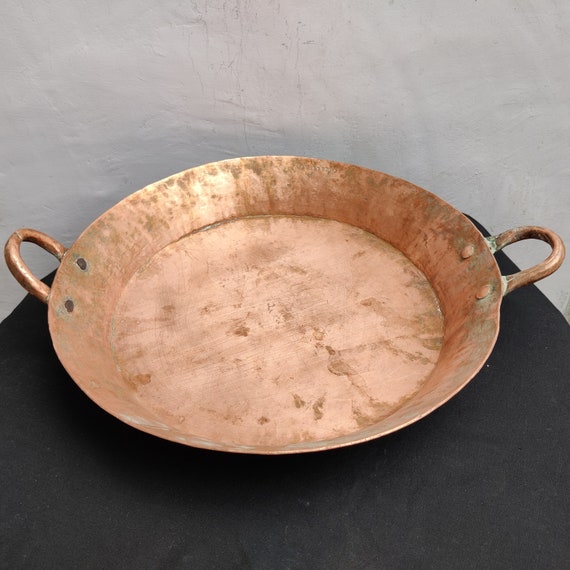The image showcases a large, rustic orange metal pan, likely made of copper or bronze, situated at the center. The pan rests on a black round surface with a grayish-white wall in the background, showing visible brush strokes. Featuring two semicircle handles on either side, the pan exhibits signs of age and wear, including various brown and dark brown markings and subtle green corrosion. The handle on the right has noticeable corrosion near the ends, while the left handle shows where buttons formerly attached have worn away, leaving rusted spots. The pan’s edges flare outward, indicating it might be used for cooking, and its handmade, dented appearance with visible brush strokes gives it an artistic and nostalgic style. Additionally, subtle details such as small round brown marks are scattered throughout the pan's surface, contributing to its rustic charm.